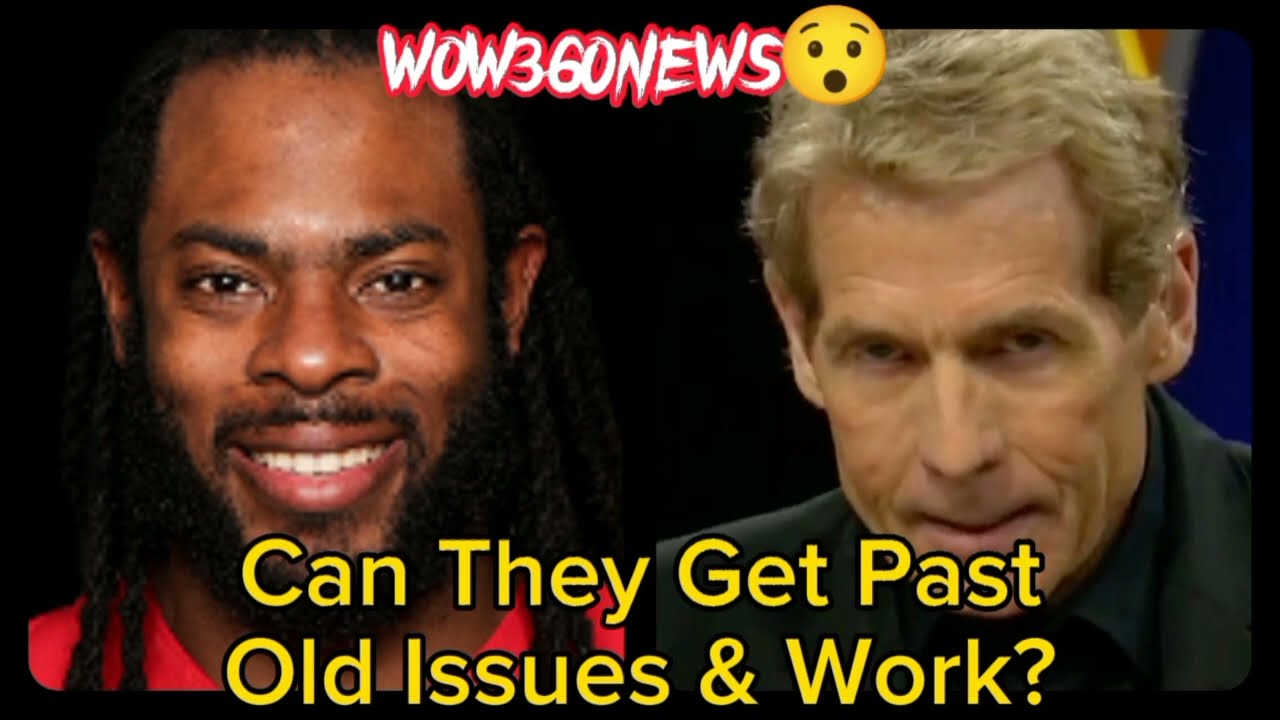The image depicts two men standing side by side, with their faces juxtaposed for contrast. At the top center, bold white letters outlined in red proclaim "Wow 360 News," accompanied by a yellow emoji face to the right, with black eyes, expressive eyebrows, and a surprised open mouth. The man on the left is a smiling black man with dark eyes, a full beard and mustache, and black dreadlocks cascading down the sides of his face. He is dressed in a red t-shirt. The man on the right, contrasting sharply, has a very fair complexion with visible wrinkles, especially on his forehead. His light brown, almost blond hair is parted on the left and appears slightly messy. He wears a black suit coat over a black button-up dress shirt, and his head is tilted downward with an angry, partially open mouth. The tension between the two is underscored by the caption at the bottom, written in bold yellow text with a black outline, asking, "Can They Get Past Old Issues and Work?"